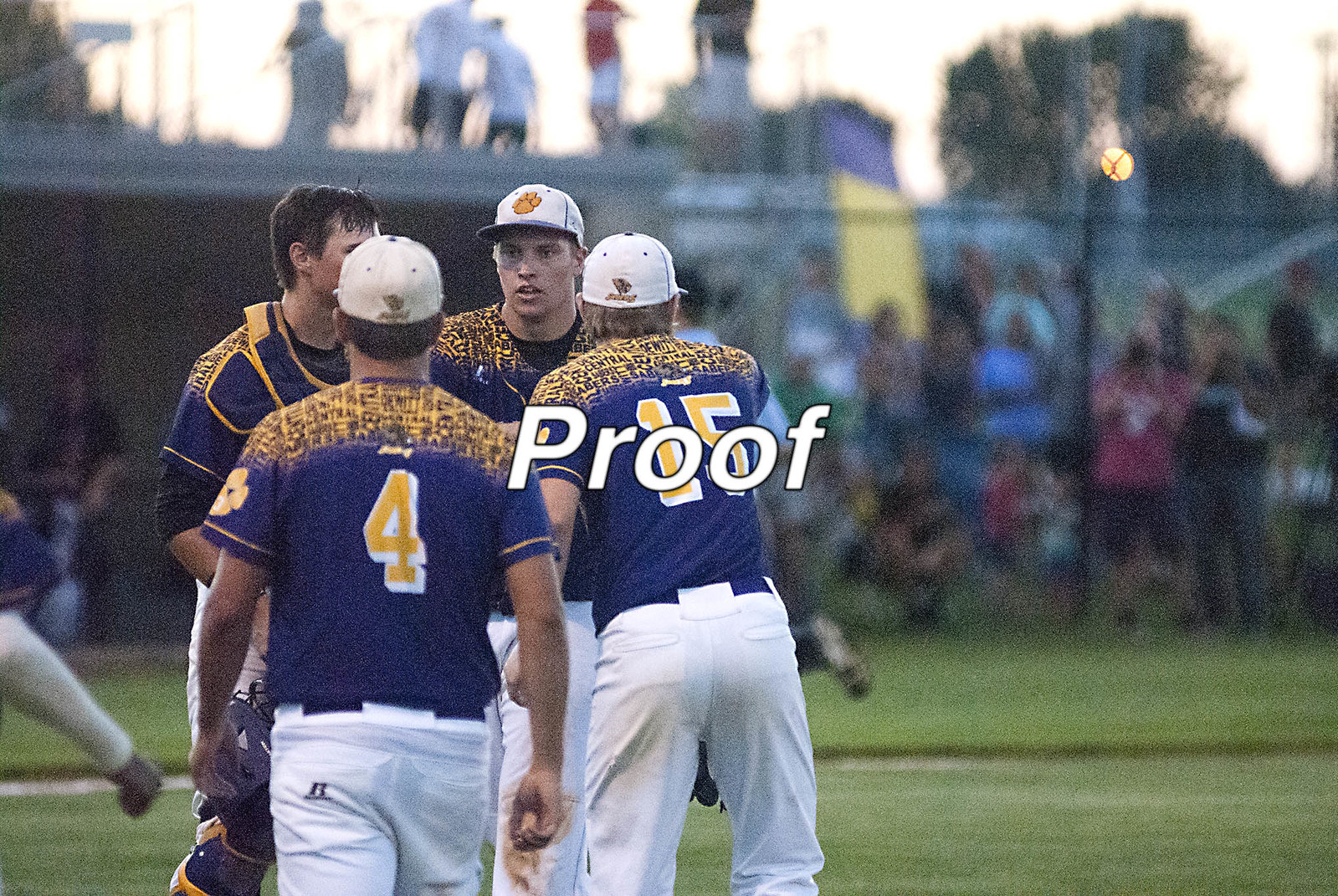This photograph captures a dynamic moment on a baseball field featuring four players in coordinated uniforms. All players are donned in white pants and blue shirts adorned with yellow sparkles on the shoulders, while the numbers on their backs are outlined in white with a yellow fill. Notably, the player on the left wears number 4, and the player on the right sports number 15. They are also wearing white baseball caps with an orange logo, except for one player who has removed his cap. The scene unfolds on a lush, forest-green grass field with a backdrop of blurred spectators behind a fence. Adding to the complexity of the scene, there is a low building visible in the background, topped by people who seem to be standing on its roof. A banner featuring purple and yellow squares is gently visible in the background. Across the forefront of the photograph is the word "proof" in white lettering.